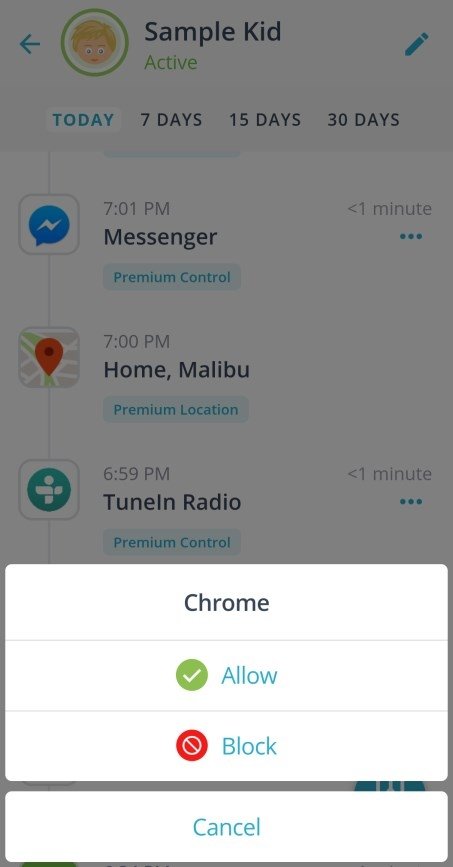The image captures a faded screenshot of what appears to be a smartphone interface. At the top of the screenshot, there is a faded gray overlay with a cyan blue arrow pointing to the left. Below this, a green circle with a dark gray border contains a profile picture. The profile picture is a cartoon-like illustration of a child with dirty blonde hair, Caucasian skin, googly black eyes, and pink lips. To the right of the profile picture, bold black text reads "Sample Kid," followed by green text indicating the status as "Active." On the far right, there is a dark blue pencil-like icon.

The interface seems to display various tabs corresponding to different periods, with the "Today" tab being selected and highlighted in blue, while the other tabs are black and set against a mid-gray background. The tabs read "Today," "7 Days," "15 Days," "30 Days," indicating time intervals.

Below the tabs is a section detailing app usage:

1. **Messenger**
   - Icon: White square with a dark gray border, containing a dark blue circle with a white lightning bolt, resembling a chat symbol.
   - Time: 7:01 PM
   - Status: "Premium Control" in a light blue rectangle with dark blue text.
   - Usage: "Less than one minute" in gray text.
   - Additional options: Three dark blue ellipses.

2. **Google Maps**
   - Icon: Dark gray with white street bands and green areas, including a red pin with a maroon circle.
   - Time: 7:00 PM
   - Location: "Home, Mali BU" in bold black text.
   - Status: "Premium Location" in a light blue rectangle with dark blue interior.
   - Usage: "Less than one minute" in gray text.
   - Additional options: Three dark blue ellipses.

3. **TuneIn Radio**
   - Icon: White square with a teal circle and white silhouette of a person.
   - Time: 6:59 PM
   - Status: "TuneIn Radio" in bold black text.
   - Usage: "Less than one minute" in gray text.
   - Additional options: Three dark blue ellipses.

Additionally, there is a pop-up at the bottom, showing app permissions for Chrome. It contains three sections with different icons and options:
- A dark green circle with a white check mark and "Allow" in blue hypertext.
- A red circle with another circle inside it, containing a line through it, labeled "Block" in blue.
- A rectangle with blue text in the center, labeled "Cancel."

The overall design suggests the interface is for monitoring or controlling app usage or permissions on a child's device.